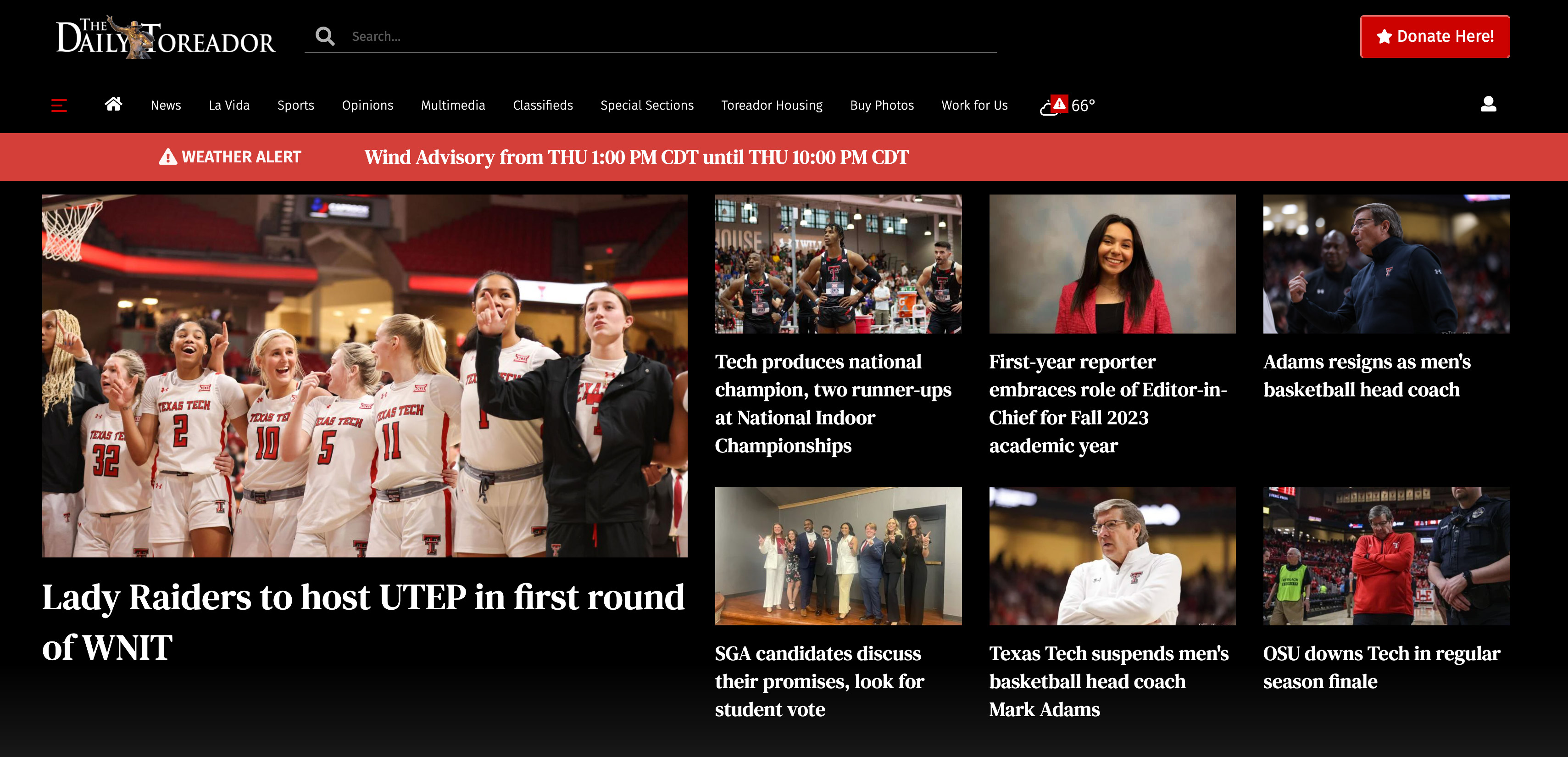Here's a detailed and cleaned-up caption for the image of the website:

---

The image showcases a webpage titled "The Daily Toreador" prominently displayed in the upper left-hand corner against a black background. On the top navigation bar, various clickable categories are available for browsing. A noticeable red "Donate Here" button with a white star is conspicuous on the page. To the right side, there is a generic profile icon.

A red bar running horizontally across the top of the screen serves as a weather alert, featuring a triangle with an exclamation point. The alert text informs users of a wind advisory valid from Thursday 1 p.m. CDT to Thursday 10 p.m. CDT.

In the main section, there's a headline and image related to the "Lady Raiders to host UTEP in the first round of WNIT," featuring a women's basketball team. Below this, six smaller images depict various sports teams, each accompanied by a brief description:
1. A girl reporter embracing the editor-in-chief.
2. Tech suspending their basketball head coach with an image of the coach.
3. Announcement of Adams resigning as men's basketball head coach.
4. A report on OSU downing Tech in the regular season finale.

Each of these images includes explicit captions to communicate the details of the events and individuals featured.

---

This caption aims to be thorough and vivid, encapsulating the webpage's content and layout without omitting critical information.